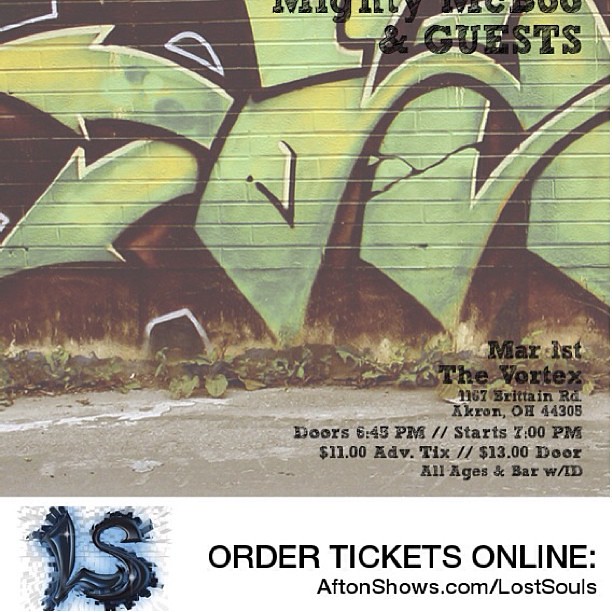The flyer for a music event features a central photograph of a brick wall covered in colorful graffiti, prominently showcasing several spray-painted arrows in green, black, and brown, pointing in various directions. The graffiti is interwoven with the readable black text, "Mighty and Guests." Below this vibrant and urban artwork, the bottom right corner details the event information: "March 1st, The Vortex, 1167 Britton Road, Akron, OH 44305, Doors 6:45 PM, Start 7 PM, $11 Advance Tix, $13 Door, All ages and bar with ID." Complementing the flyer’s artistic design, the bottom left corner features a creatively drawn blue logo with the letters "LS" and instructions to order tickets online at aftonshows.com/lostsouls. The lower part of the image reveals the ground with a cemented floor, scattered leaves, and bits of trash, adding to the raw, authentic vibe of the event’s promotion.